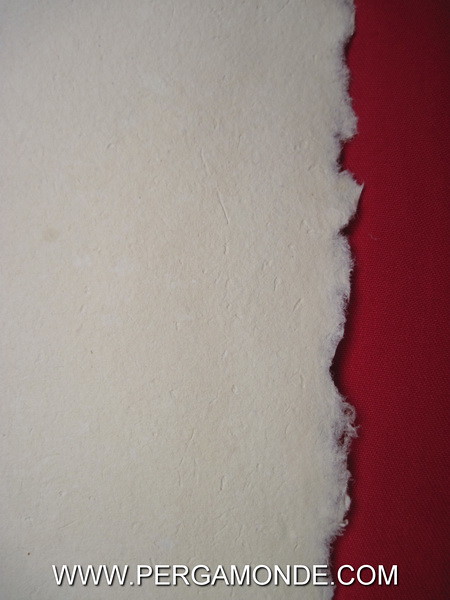The photograph captures a dynamic contrast between two distinct textures and colors. Dominating the left side of the image, a white, furry material with irregular, torn-like edges lies over a rich, red, cloth-like surface that occupies the right side of the frame. The furry white fabric displays numerous markings and scratches, adding to its textured appearance. At the bottom middle of the image, the URL "www.pergamond.com" is prominently displayed in bold white text, outlined in black for emphasis, completing this visually striking composition.